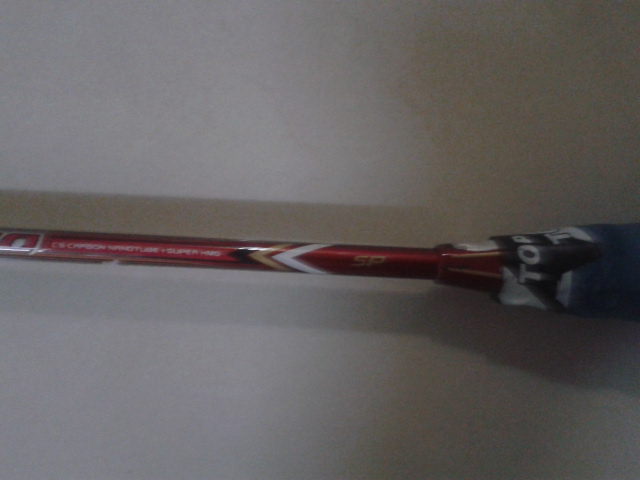The photograph captures an indoor scene featuring a long, thin object positioned horizontally against a grayish-white background. The object resembles a tube or pole, possibly related to sporting equipment like a ski pole or racket. Stretching from right to left, the object is characterized by a thicker handle on the right side, which is primarily blue, accented with white and black. On this handle, the white letters "T.O.P." are prominently displayed. The main shaft of the object is slender, predominantly red, with patterns in white, black, beige, and gold. In the center of the shaft, the gold letters "S.P." are visible, and further along the shaft, smaller, illegible writing is faintly discernible. The object casts a shadow behind it, adding depth to the image.